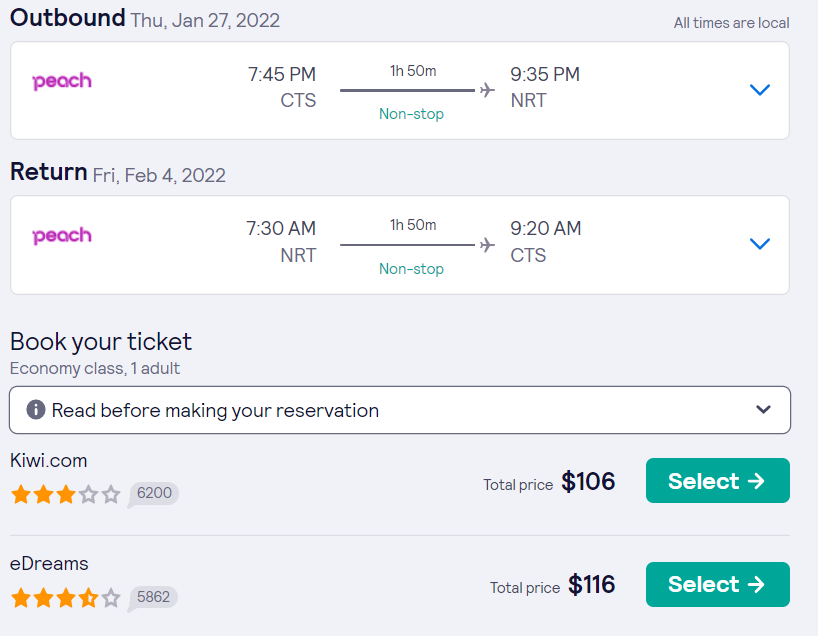The image is a detailed screenshot of an airline ticket booking page, showcasing information for an outbound flight and a return flight. The outbound flight is scheduled for Thursday, July 27, 2022, while the return flight is set for Friday, February 4, 2022. Both flights are non-stop and have a flight duration of one hour and fifty minutes.

At the top of the screenshot, the departure and arrival times for both flights are clearly indicated. In the center of the image, there is an option to book tickets for one adult in economy class. 

The lower section of the screenshot features two different websites from which the tickets can be purchased: Kiwi.com and eDreams. Kiwi.com offers tickets priced at $106 with a rating of three stars out of five based on 6,200 reviews. eDreams, on the other hand, has tickets priced at $116 and boasts a slightly higher rating of 3.5 stars, derived from 58,862 reviews.

At the very bottom, there are options to choose either of the websites for finalizing the ticket purchase.